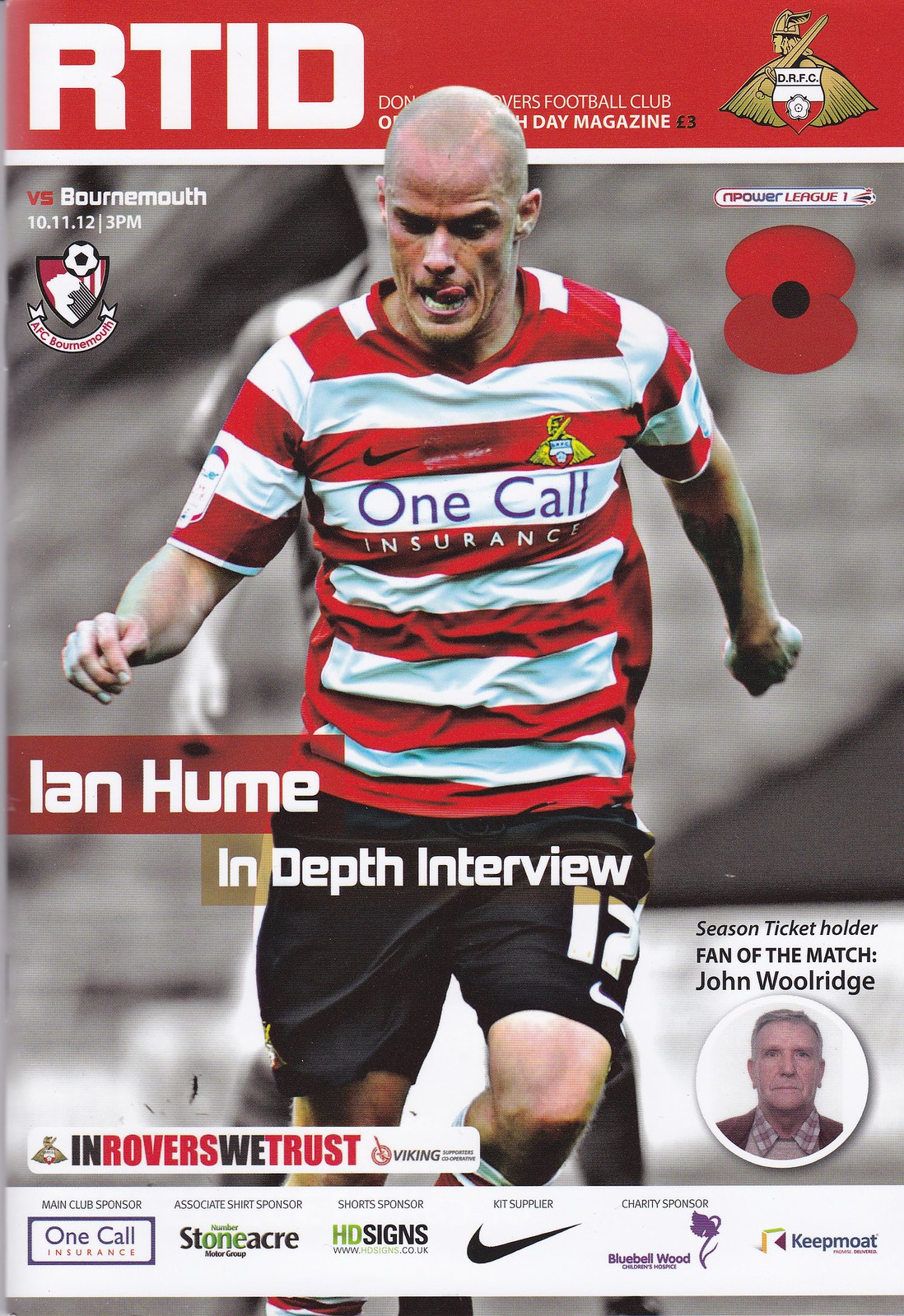A vibrant poster advertises a football match, highlighting an in-depth interview with player Ian Hume. The top of the poster features a red background with white letters reading "RTID," and to the right, it says, "Doncaster Rovers Football Club Magazine," accompanied by the club's logo. Below this, the crucial detail stands out: "versus Bournemouth, 10-11-12 at 3 p.m."

The central image showcases Ian Hume, clad in a red and white striped jersey bearing the "One Call Insurance" logo across the central white stripe, and black shorts with the number 17. Hume, seemingly of Hispanic descent, is captured in motion, looking down at the ground in a running position. Next to him, the text proudly announces, "Ian Hume, In-Depth Interview."

At the bottom, a black and red banner declares, "In Rovers We Trust," flanked by various sponsor logos including Nike, One Call Insurance, Stoneacre, Keepmoat, and HD Signs. In the lower right corner, a special nod is given to season ticket holder John Wooldridge, named as the "Fan of the Match," with his circular photo displaying below the title.

The overall color scheme predominantly features red, white, and black, punctuated by sponsor logos and other text, creating a dynamic and engaging visual.